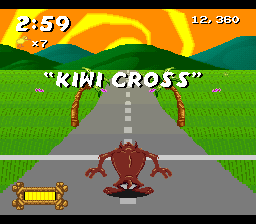A screenshot from a video game is shown with a square frame featuring black bands at the top and bottom. The upper background is primarily orange, accented by three curves of arching yellow lines that suggest a sunrise. The time displayed is "2:59," with additional data "time 7" beneath it and "12,360" on the opposite side. Below the sun, rolling mountains in alternating green and blue hues stretch across the screen. A straight, two-lane road with intermittent dashed lines divides two grassy sections. The words "Kiwi Cross" are enclosed in quotation marks above the road. Alongside the road, there are two brown arches. In the foreground, a brown, reptilian creature with a menacing appearance stands facing the road; its tail is visible behind it, and it has pointy appendages that seem to be ears, a thick torso, and slender limbs. In the bottom left corner, a yellow rectangle with a gold trim adds an additional dash of color.